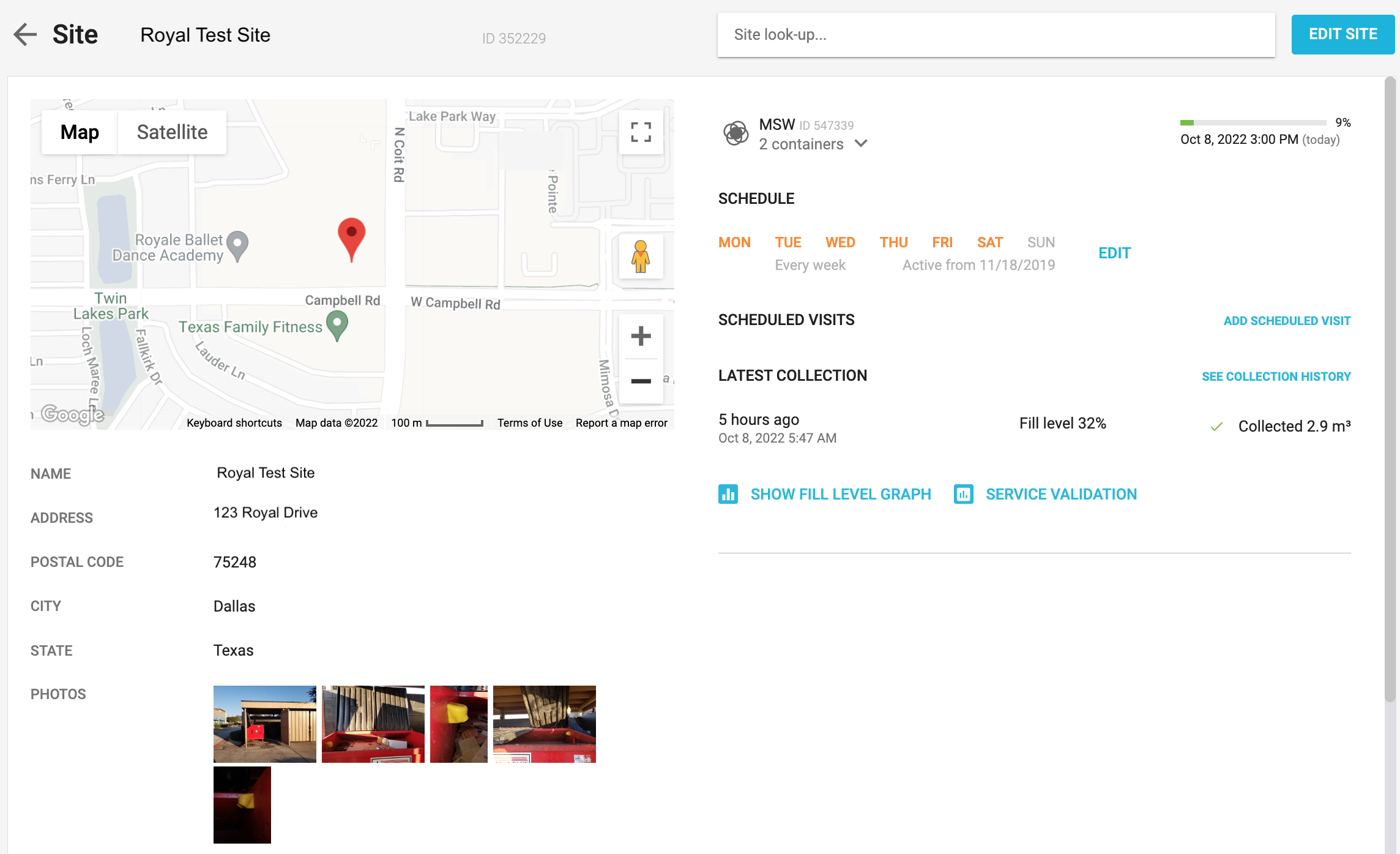This screenshot captures the interface of a website titled "Royal Test Site." In the upper left corner, the website features the word "Site" and a left-pointing arrow. The search bar, labeled "Site Look Up," sits prominently below, alongside a blue "Edit Site" button in the upper right corner.

At the center of the page, there's an image of a map. The map is predominantly in dark black with a satellite or lighter black view, showing a street map with a pinpoint marking the location of the Royal Test Site. Beneath the map, the site’s name, "Royal Test Site," is clearly listed along with its address in Dallas, Texas. 

On the right side of the page, a segment titled "MSW Two Containers" includes a drop-down menu for selecting schedules. The schedule runs from Monday through Saturday, with Sunday left blank, which users can edit. There are options to add new schedules and review the latest collection data, both highlighted in blue. Historical collection data from five hours ago shows fill levels at 32%, with 2.9 million units collected. Additionally, users can access a fill level graph and service validation features.

Below the map, a gallery of five photos showcases the exterior of the Royal Test Site, with dominant colors being red and brown. There may also be images of the interior. The interface provides a comprehensive overview of the site’s operational details and features.